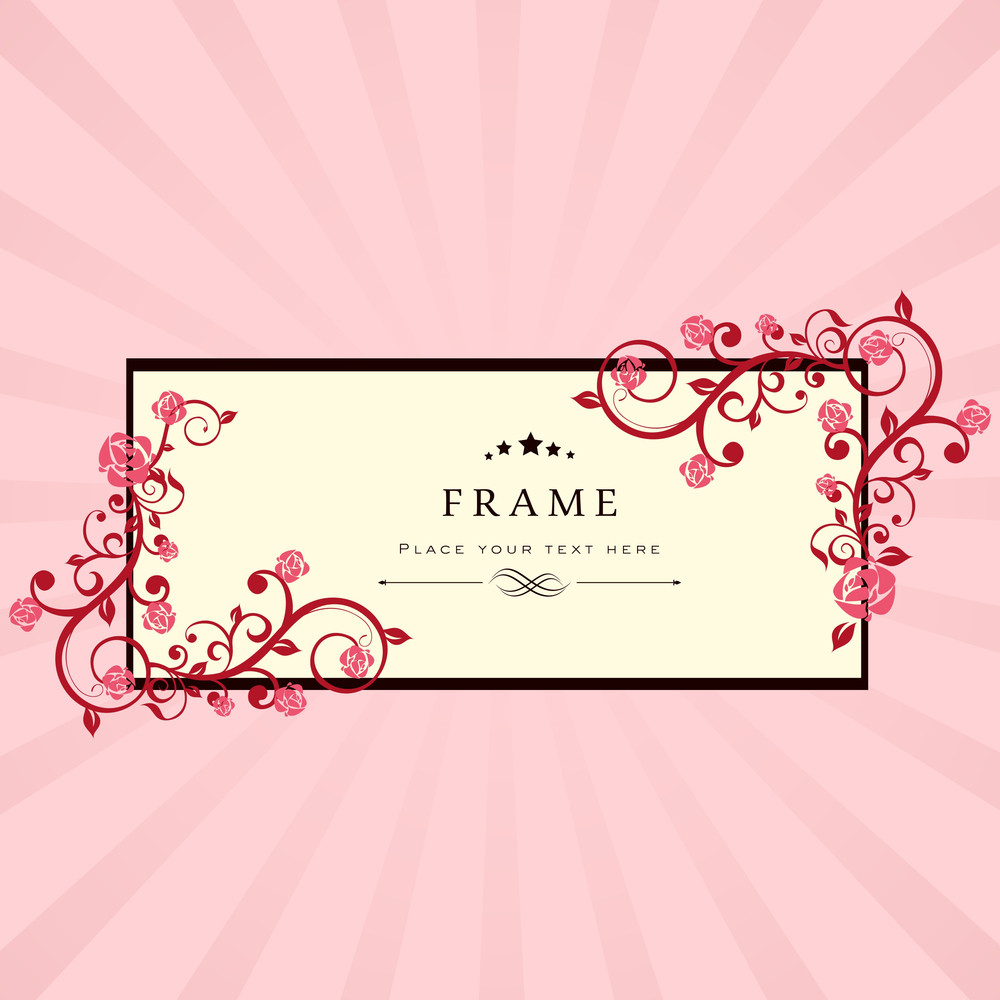The image presents a detailed and ornate clipart template suitable for various purposes, such as printing or email messages. Dominating the background is a rose-colored sunburst pattern that varies from light pink to dark pink, creating a radiant effect that draws the eye to the center. Over this background lies a cream-colored horizontal rectangle with a solid black border. 

Inside this frame, at the top, is an arc of five stars with the one at the center being the largest. Below the stars, the word "FRAME" is displayed prominently in all caps and a spaced-out serif font. Just beneath it, in all caps and a sans serif font, is the placeholder text "PLACE YOUR TEXT HERE." Further down, there are two arrows pointing towards the edges with an ornate figure-eight shape between them.

The rectangle is further adorned with intricate scroll designs featuring roses and leaves in the lower left-hand and upper right-hand corners. These elements consist of a combination of dark red and slightly lighter rose tones, giving the design an elegant and sophisticated floral touch.